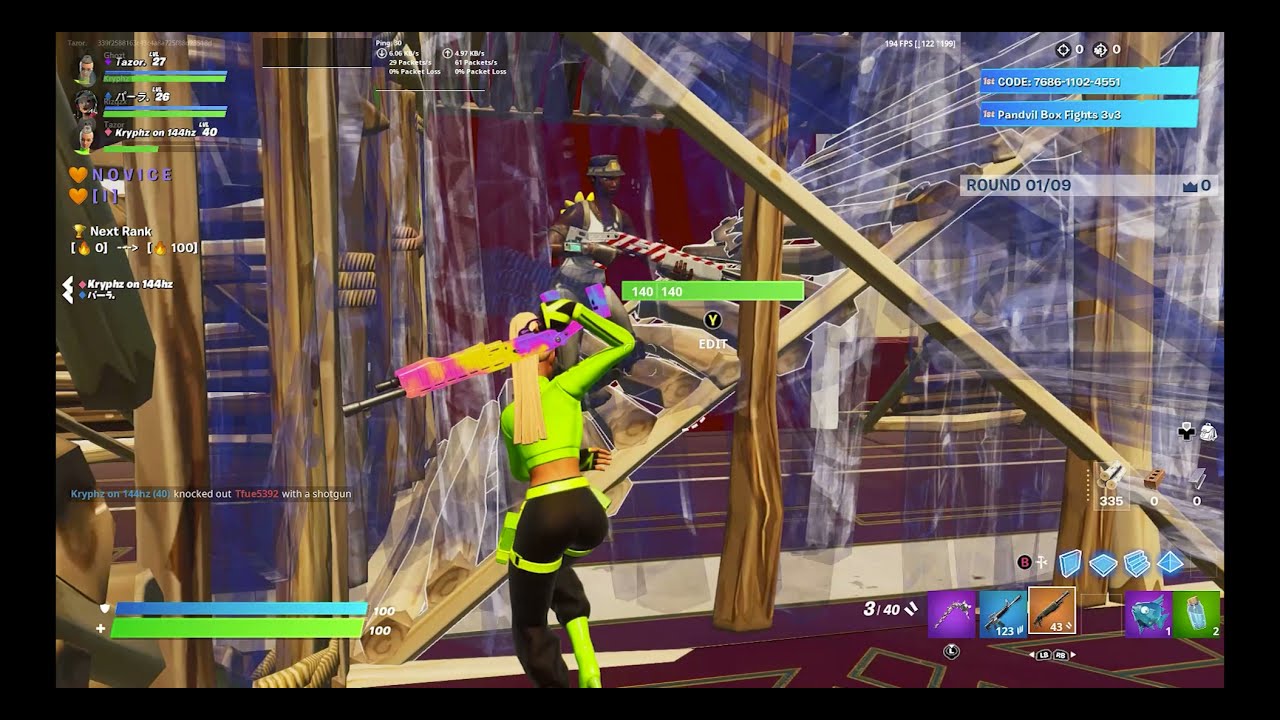The image is a detailed screenshot from the video game Fortnite, showcasing two characters in the midst of an action scene. Centered in the image is a female character with dark skin, sporting a unique appearance featuring blonde hair tied back in a ponytail that reaches halfway down her back. She is dressed in a cropped, neon green jacket with black stripes, black pants with matching neon green accents, and lime green boots. Around her waist is a lime green belt, and she wields a large, brightly colored rifle in shades of purple and yellow.

Accompanying her is another male character, also with dark skin, who appears to be wearing a dark hat and a muscle tank top. He holds a red and white striped gun, reminiscent of a candy cane. The background reveals they are ascending wooden stairs, seemingly constructed from light brown wood, with some blue glass walls. Above them, the game's HUD is visible, indicating weapons, ammo, health, and armor stats. Notable HUD details include round information (Round 1 of 9), character and player names, and various icons such as an orange heart, gamer tags, health bars (blue and green at 100%), and fire symbols.

The scene is vibrant with a blend of colors including green, black, brown, maroon, blue, red, purple, and orange, reflecting the game's lively and detailed design. The characters appear to be on a mission with their distinctive weapons, underscoring the dynamic and engaging environment of Fortnite.